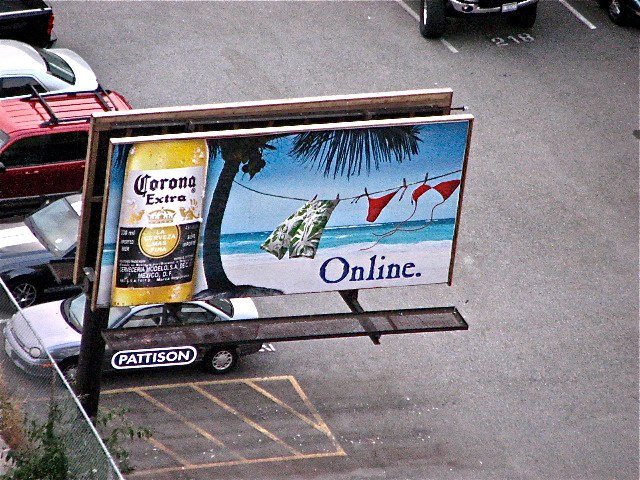Captured from an elevated vantage point, possibly from a tall building or a drone, this image showcases a bustling parking lot with several cars parked in an orderly fashion. Notably visible are a silver sedan, a blue car with a distinctive white stripe, a red SUV, and another silver car in the distance. The central focus of the image, however, is a large billboard owned by Pattinson, prominently placed at the base of the frame. The advertisement on the billboard features a vibrant promotion for Corona Extra. On the left side, there's a refreshing image of a Corona Extra bottle beside a picturesque palm tree. Extending from the palm tree, a clothesline drapes across the scene, adorned with colorful men's and women's bathing suits fluttering in the breeze. The background of the billboard is a serene depiction of a sandy beach meeting the tranquil ocean, altogether evoking a summery, tropical vibe.